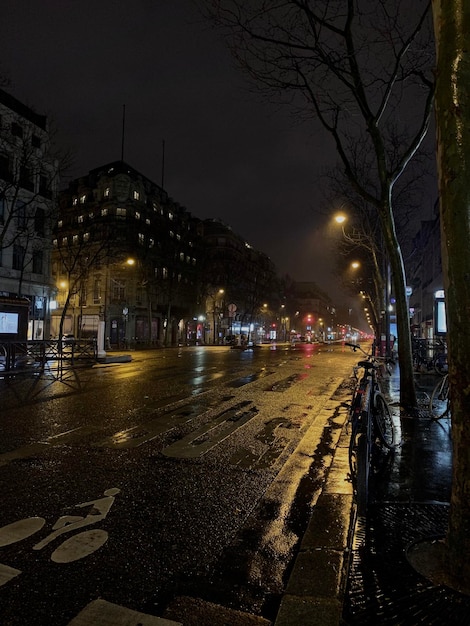This image captures a serene, rainy night in a town or city. The night sky, tinged with deep blue and gray hues, appears slightly cloudy, creating a dreamy backdrop. The wet roadway glistens under the yellow shine of street lights, giving it a golden-brown tint in certain areas. This road, featuring a cycling lane marked with a bicycle decal, shows minimal traffic, and there are stop signs and other road markings visible. Multi-storied buildings with storefronts at the bottom line both sides of the street, some windows illuminated, hinting at lingering activity, while others remain dark, possibly offices emptied for the night. On the right-hand side, a sidewalk accommodates several trees, which are bare and bicycles parked beside them. The scene, devoid of bustling activity, exudes a calm, post-rain charm, with every element bathed in the tranquil glow of the street lights.